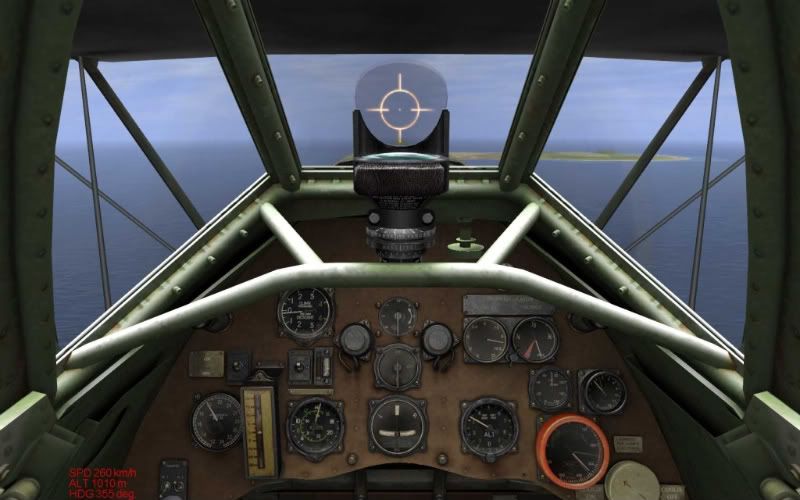This photograph captures the interior of a vintage military aircraft cockpit, characterized by the surrounding metal framework and an array of gauges and monitors, resembling watches, displaying various indicators such as speed, altitude, and temperature. Prominently, an illustration of a targeting crosshair is visible at the center of the cockpit window, possibly representing the pilot's view. The view outside the cockpit reveals a vivid scene of a blue ocean, a clear blue sky, scattered clouds, and a narrow green strip of land that appears to be an island. The image includes a watermark with the logo and name "Photobucket" positioned mid-center, accompanied by the promotional slogan "Protect more of your memories for less" in black text with a gray rectangular border beneath it, suggesting an advertisement for the Photobucket service.